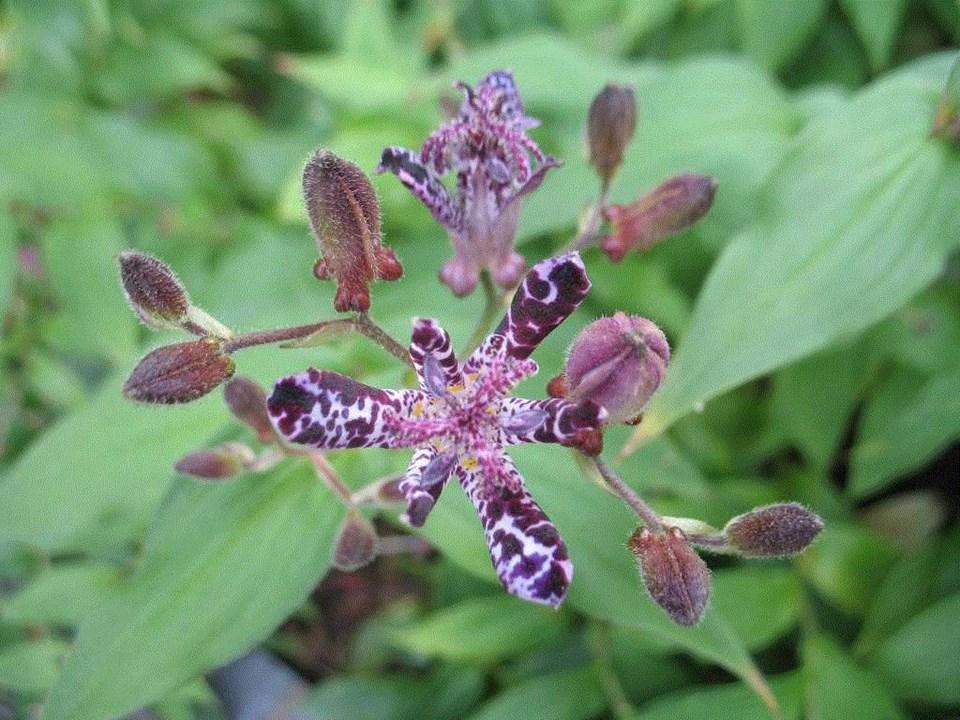This photograph captures a striking botanical scene with a blurred background of green leaves, some showing yellow-brown spots and others appearing crisp and healthy, creating a painterly effect. In the foreground, there are two prominently detailed flowers that could be orchids due to their intricate structure and exotic beauty. The foremost flower is angled towards the viewer, displaying three large, white petals adorned with dark purple spots and three smaller petals with a matching color scheme. From its center, three pink tendrils curve outward in different directions. The second flower, slightly behind, has pink and purple petals that arch upwards and outwards, with a burst of drooping tendrils springing from its center. Surrounding these blossoms are several unopened buds, covered with fine hairs and a dark purple and green hue, positioned thoughtfully around the flowers—three up and to the left, three blurred down and to the left, two down and to the right, and two blurred up and to the right. The lighting appears to be natural daylight, suggesting this scene was captured in someone's garden or in the wild, where these flowers thrive amidst a lush tapestry of foliage.